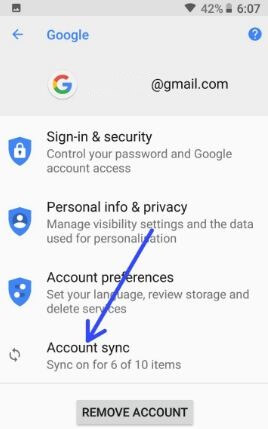The screenshot on the phone displays a battery level of 42% and a time of 6:07. Below this, there is a gray box featuring a blue arrow pointing left, the word "Google" in blue text, and a blue circle with a question mark inside. Directly under this, to the left, there is a white circle with a rainbow-colored 'G' in the middle, representing the Google logo. Next to this logo, black text reads "I'm at gmail.com." 

Below these elements, on a white background, there is a shield icon with a lock in the center. Accompanying this icon, black text reads, "Sign-in & security," and in gray text, it states, "Control your password and Google account access."

Further down to the left, there is a blue shield with a silhouette of a person. Next to this, black text says, "Personal info & privacy," with gray text below stating, "Manage visibility settings and the data used for personalization."

Finally, beneath that section, there is another blue shield icon featuring two microphones. Adjacent to this, black text reads, "Account preferences," and gray text beneath it states, "Set your language, review storage, and delete services."